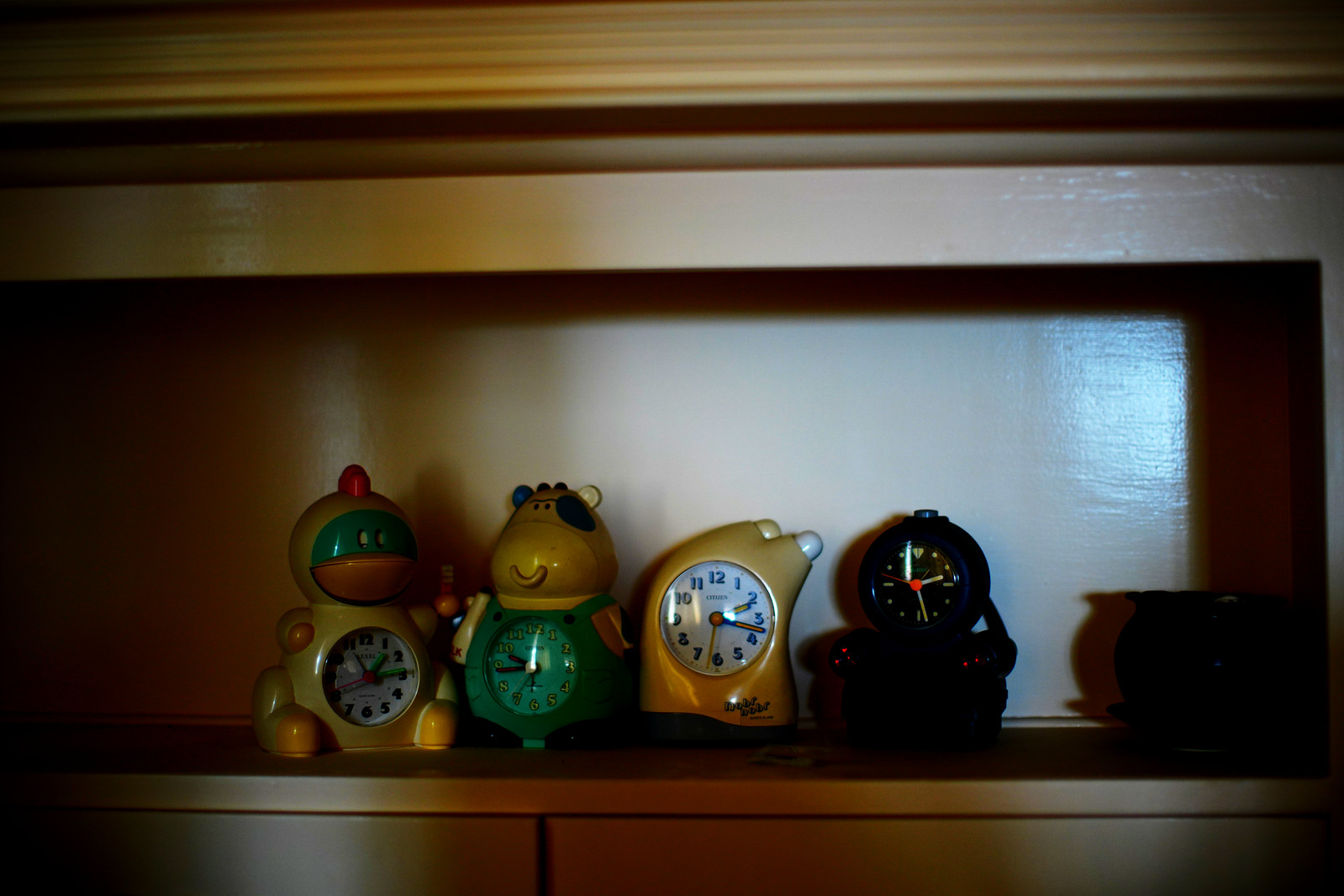This photograph features a collection of four novelty clocks displayed on a brown wooden shelf within a bookcase or cabinet against a white wall backdrop. The first clock on the left resembles a duck with a yellow body, orange beak, red mohawk-like ridge, and a green face. The white clock face with green hands is located on its belly. Next to it is a golden cow figurine with black spots, green overalls, and a green clock face with black hands situated on its belly. The third clock has a unique design, resembling a pair of bananas, sporting a gold color with a curved pattern to the right, marked by two white buttons on the side and a white clock face with blue numbering. The final clock on the right is black and circular, mounted on a dark, possibly rectangular base that blends into the shadows, making it difficult to discern. The scene is somewhat dimly lit, adding a shadowy quality to the overall image.